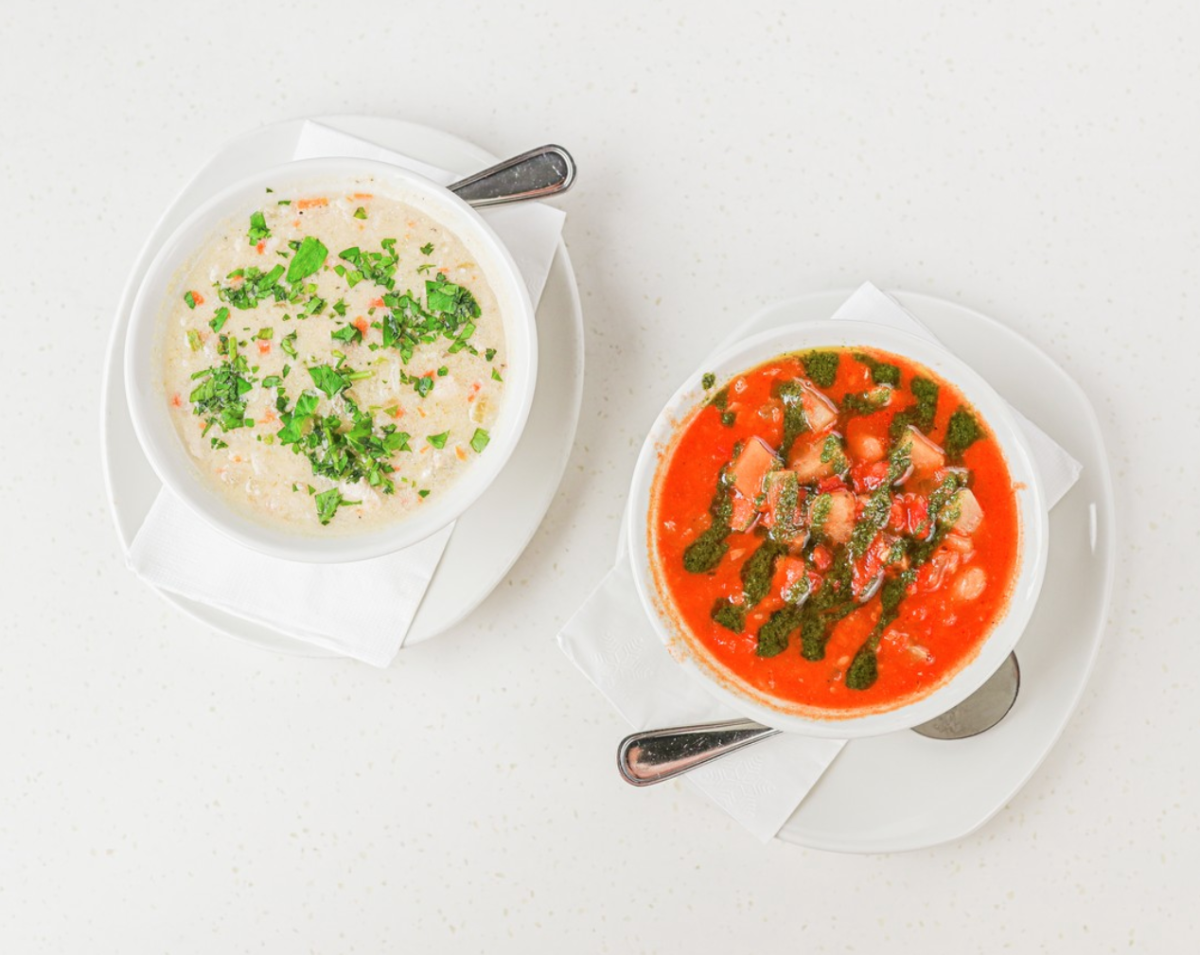The image depicts a professional, top-down photo of two bowls of soup on a mostly flat white surface with faint grey speckles. Each bowl is placed on a rectangular white napkin and an oval-shaped white plate, accompanied by a silver spoon positioned on the plate. On the left side, slightly above center, there's a circular white bowl containing a creamy, whitish soup accented with green herb sprinkles and bits of orange, likely pieces of vegetables or seasoning. On the right side, slightly below center, another white bowl features a vibrant red tomato-based soup with a green sauce drizzled in a striped pattern and chunks of vegetables or other ingredients. The presentation is meticulous and visually appealing.